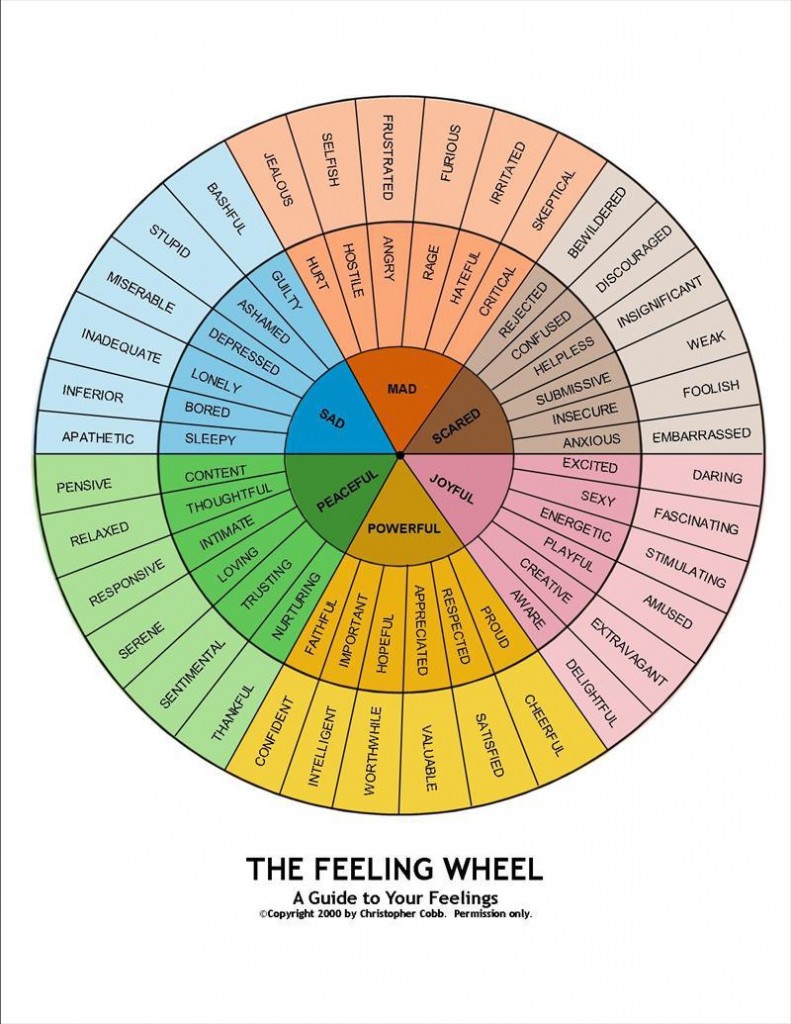The image is a detailed and colorful diagram known as "The Feeling Wheel," created by Christopher Cobb in 2000. It features a large outer circle with two nested inner circles, culminating in a smaller central circle divided into triangular sections. The inner circle segments the wheel into primary emotions, each marked by distinct colors and placed at strategic positions around the wheel.

Starting from the 12 o'clock position and moving clockwise, the primary emotions are as follows: "Mad" (in red), "Scared" (in brown), "Joyful" (in pink), "Powerful" (in mustard yellow), "Peaceful" (in green), and "Sad" (in blue). 

Each of these primary emotions further branches out to secondary emotions, providing a more granular representation of feelings. For example, under the primary emotion "Joyful," the secondary emotions are "Excited," "Sexy," "Energetic," "Playful," "Creative," and "Aware." These secondary emotions then extend to tertiary emotions, such as "Daring," "Fascinating," "Stimulating," "Amused," "Extravagant," and "Delightful."

This wheel serves as a comprehensive guide to understanding and identifying a broad range of human emotions, offering insights into how primary feelings can evolve into more specific emotional states.